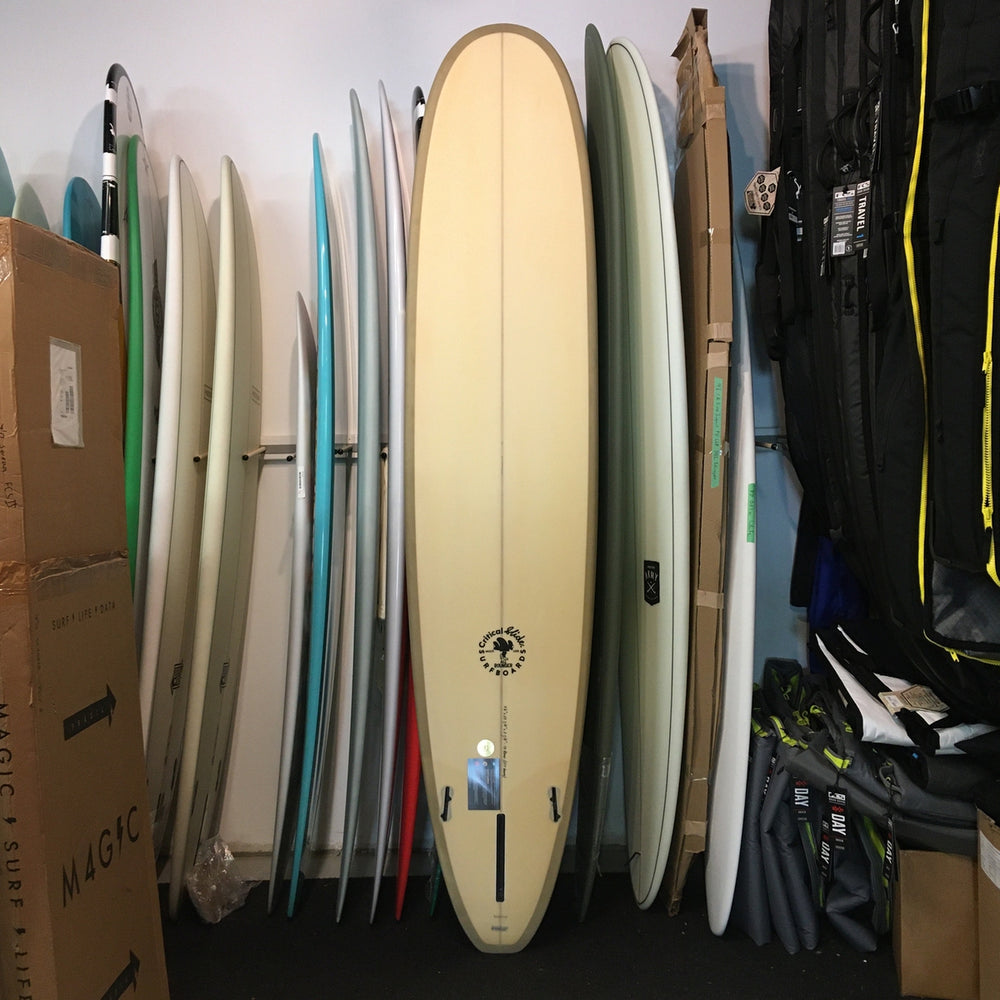The photograph captures a storeroom, likely within a surf shop, featuring an array of surfboards neatly organized in a rack. Most of the surfboards are standing sideways, displaying a variety of colors, including yellow with a tan outline, green, gray, aqua, and several in white. One prominent beige surfboard stands front-facing against the white wall, which sets a plain backdrop for the vivid array of boards. The boards range in sizes from small to traditional lengths, catering to different surfing needs. In addition to surfboards, the room contains numerous cardboard boxes, one prominently marked with "M4GIC" alongside an arrow. There are also garment bags and what appear to be wetsuits hanging to the right. Various other items, possibly backpacks with tags, rest atop some boxes, emphasizing the multipurpose nature of this storeroom dedicated to surfing paraphernalia.